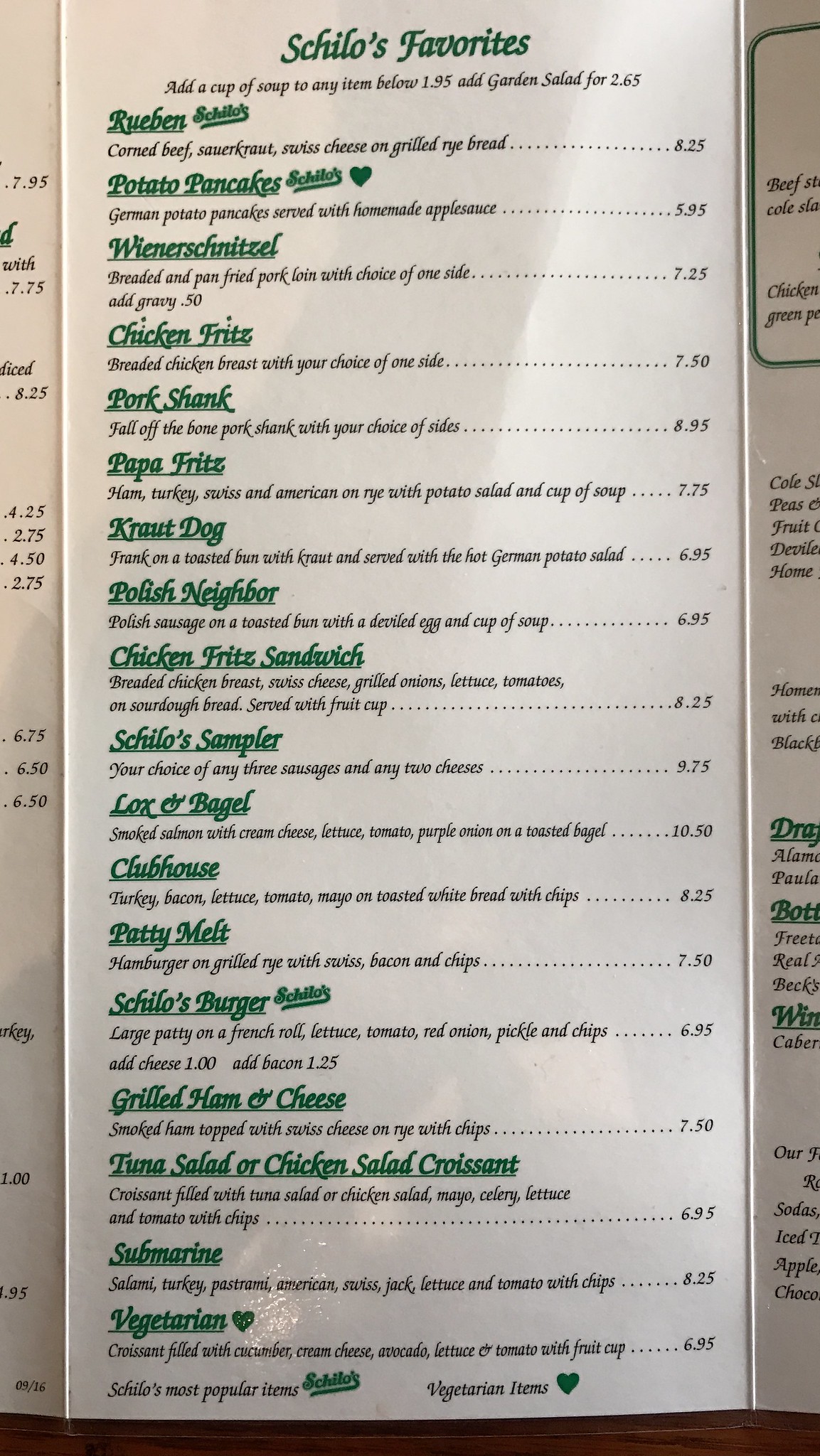**Menu: Ski-Lo's Favorites**

- **Add-ons**:
  - Cup of soup: $1.95
  - Garden salad: $2.65

1. **Reuben Sandwich**:
   - Corned beef, sauerkraut, Swiss cheese, on rye bread
   - Price: $8.25

2. **Potato Pancakes**:
   - Served with shrimp and homemade apple pie
   - Price: $5.95

3. **Wiener Schnitzel**:
   - Breaded and pan-fried pork loin with one side
   - Price: $7.25
   - Add gravy: $0.50

4. **Chicken Fries**:
   - Breaded chicken breasts with three sides
   - Price: $7.50

5. **Pork Shank**:
   - Pork shank with sides
   - Price: $8.95

6. **Apple Fries**:
   - Ham, turkey, Swiss, and American cheese with potato salad and a cup of soup
   - Price: $7.75

7. **Hot Dog**:
   - Served with an egg on a bun
   - Price: $6.65

8. **Poached Neighbor**:
   - Pork sausage and a bun with a dollop of egg and a cup of soup
   - Price: $6.65

9. **Chicken Breast Sandwich**:
   - Breaded chicken breast, schnitzel skewers, breaded onions, lettuce, tomatoes, on salad bread served with fruit salad
   - Price: $8.25

10. **Yellow Sampler**:
    - Choice of any three sausages and any two cheeses
    - Price: $9.75

11. **Lox and Bagel**:
    - Smoked salmon with cream cheese, lettuce, tomato, purple onion, on a toasted bagel
    - Price: $10.55

12. **Turkey BLT**:
    - Turkey, bacon, lettuce, tomato, mayo, on a bun
    - Price: $10.25

13. **Freddie Mac Burger**:
    - Hamburger with grilled rye, Swiss cheese, bacon, and chips
    - Price: $7.50

14. **Scoops Burger**:
    - Large patty, French roll, lettuce, tomato, red onion, pickle, and chips
    - Price: $6.75
    - Add cheese: $1.00
    - Add bacon: $1.25

15. **Grilled Ham and Cheese**:
    - Smoked ham topped with sweet cheese, on rye with chips
    - Price: $7.50

16. **Tuna Salad Croissant**:
    - Croissant filled with tuna salad, mayo, celery, lettuce, and tomato
    - Price: $6.75
    - Chips: $8.25

17. **Salami, Turkey, and Pastrami Sandwich**:
    - Salami, turkey, pastrami, lettuce, and tomato with chips
    - Price: $8.25

18. **Vegetarian Croissant**:
    - Croissant filled with ketchup and cream cheese, avocado, lettuce, and tomato with fruit salad
    - Price: $10.25

19. **Skittles**:
    - Most popular item
    - Vegetarian option
    - Note: Part of the menu is cut off at the edges, so additional items may be present.

(Note: This menu seems to be undated and has some items that might need clarification or correction, such as 'skittles' and menu semantics.)